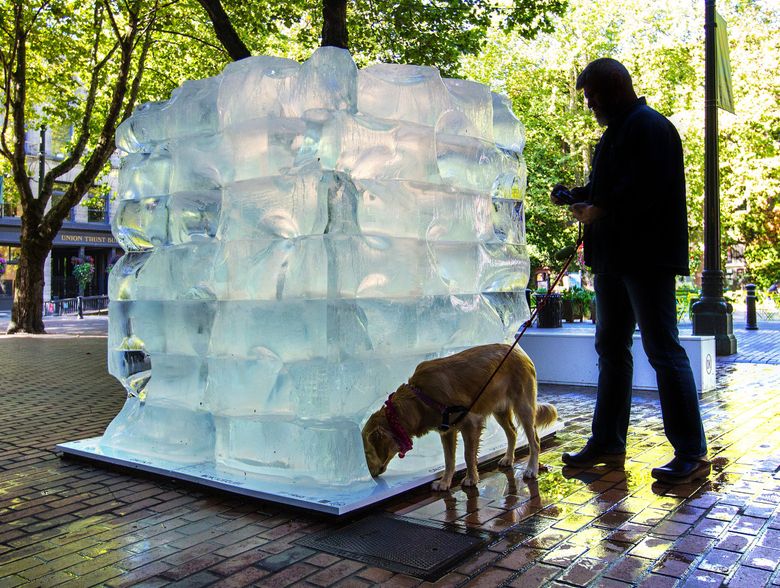This photograph captures a serene moment in what appears to be the central area of a town's shopping district. At the heart of the scene is a striking ice sculpture, composed of several rectangular blocks of ice, stacked together to form a structure that stands nearly as tall as the man next to it — approximately five and a half to six feet. The sculpture rests on a white, metal platform, set on a cobblestone or brick-paved surface.

The scene appears to be in early spring, indicated by the trees full of green leaves and the man’s jacket, suggesting a chill in the air. Surrounding the sculpture are various elements of urban life — mature trees, black lamp posts, a fire hydrant, and what look to be shops and restaurants lining the street. The atmosphere hints at a park area nestled within the urban setting, complete with places to sit and pathways.

The man in the photograph is dressed in a dark coat, blue jeans, and brown shoes. His face is slightly obscured, either due to lighting or the angle of the shot, but he appears to have a beard and short hair. He stands patiently, holding a brown leather leash attached to a golden Labrador Retriever with a red bandana around its neck. The dog is noticeably fixated on the melting ice, perhaps sniffing or attempting to drink from the pooled water on the wet cobblestones. The image captures a juxtaposition of the ephemeral ice sculpture against the vibrant, green, and seemingly perpetual elements of the town, framed by urban architecture and daily life.